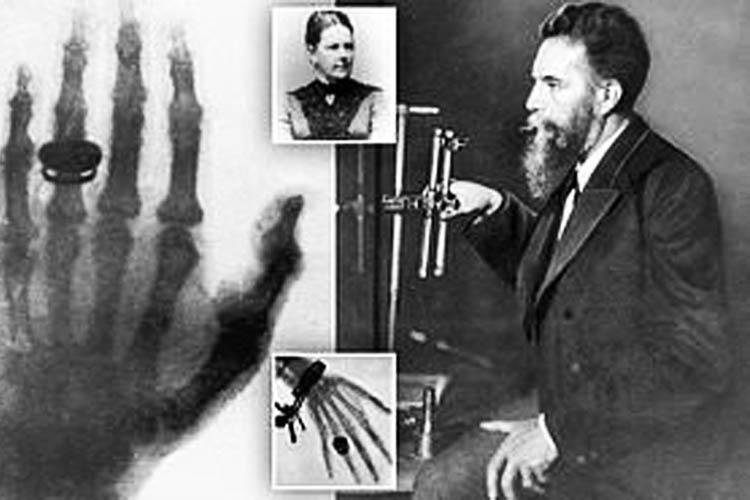This black and white vintage photograph, likely from the late 1800s to early 1900s, captures one of the earliest demonstrations of x-ray technology. In the center of the image stands a woman dressed in period attire, while a bearded man, identified as scientist Wilhelm Röntgen, operates an unclear device on the right. On the left side, an x-ray image of a left hand adorned with a ring and bracelet is prominently displayed. Additionally, a smaller inset photograph shows another x-ray, presumably of the same woman's hand. This historic scene showcases Röntgen's pioneering work with x-rays.